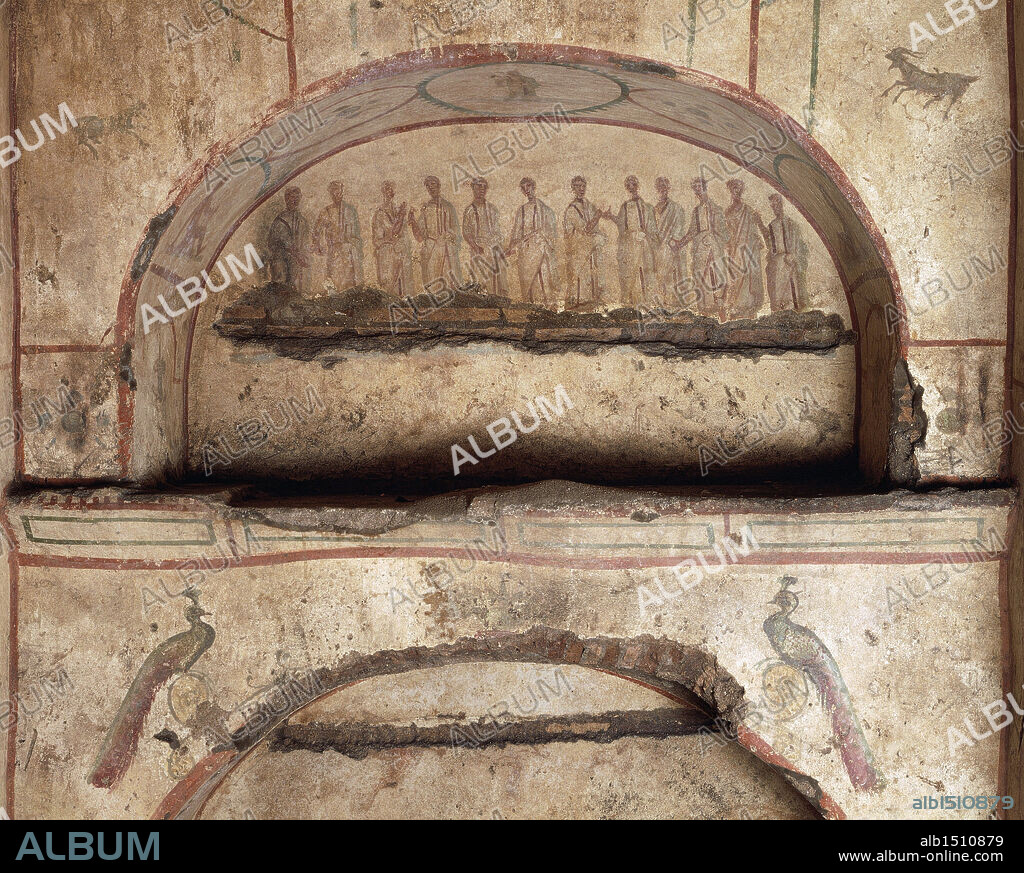This photograph captures an interior section of a mausoleum adorned with ancient Grecian or Roman artwork. Dominating the scene is a large, arched structure featuring twelve robed figures, possibly apostles, depicted in various poses, some with arms raised, all gazing downward toward a dirt-covered area. Above these figures, the arch is decorated with intricate paintings, including a distinctly visible peacock on each side with their tails down, not fanned out. An additional depiction of a ram can be found in the upper right corner of the arch. Beneath this tableau, there is a shelf outlined in faded red, supporting further artistic elements. The entire stone surface has a pinkish hue, contributing to its ancient ambiance. The photograph bears a watermark saying "album" and includes a black banner at the bottom with additional text and web address: www.album-online.com.